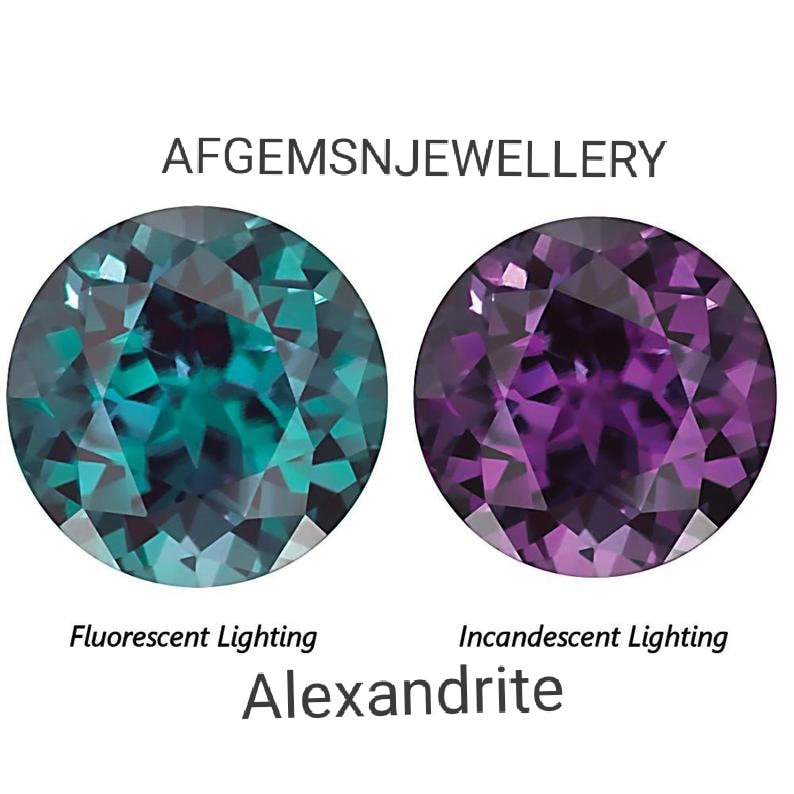This image features a detailed, graphical representation of two rounded gemstones, each depicted with geometric shapes, mainly triangles. Displayed on a clean white background, the top portion of the image contains the title "AF GEMS AND JEWELLERY" in bold black capital letters. Centrally, the image showcases two large circular gemstones side by side. 

The gemstone on the left is a rich green color with hints of black throughout and is labeled underneath as "fluorescent lighting." This gemstone also features intricate geometric patterns. The gemstone on the right is a vibrant purple with scattered touches of black and lighter purple shades at the bottom, labeled "incandescent lighting." Both gemstones exhibit a translucent quality, resembling facets of a diamond, giving them a cubist-like appearance.

Centered at the bottom of the image, the word "ALEXANDRITE" in bold capital letters indicates that these gemstones emulate the appearance of the rare and valuable material known for changing color under different lighting conditions.